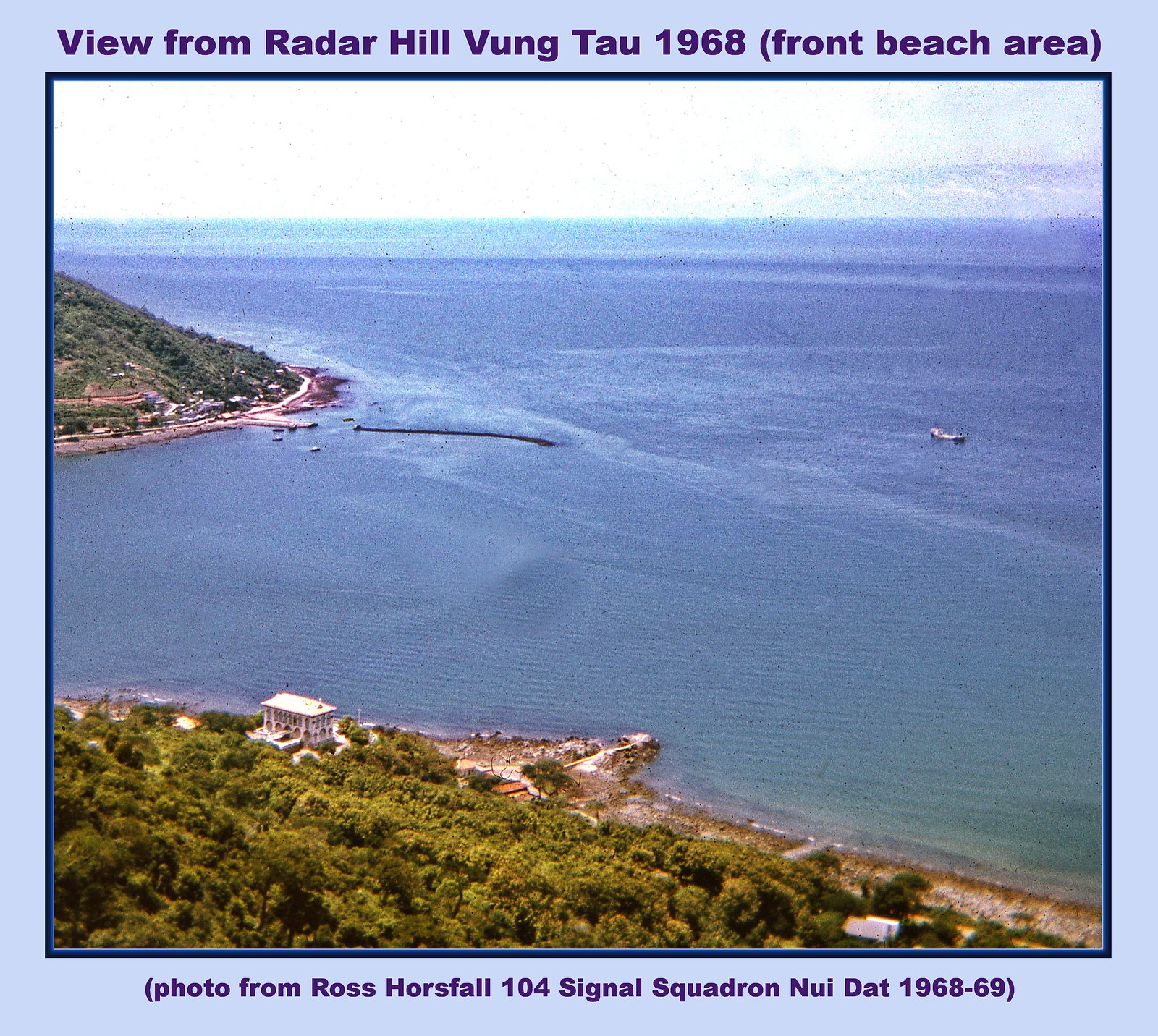The image is a color outdoor daylight photograph of an ocean scene taken from the vantage point of Radar Hill in Vung Tau, 1968. This scenic view captures the front beach area with a blue border framing the picture. The top of the image has purple text that reads, "View from Radar Hill, Vung Tau, 1968," while the bottom text states, "Photo from Ross Horsfall, 104 Signal Squadron, Nui Dat, 1968-69." 

The foreground shows a heavily forested hill descending away from the photographer, leading to a shoreline with buildings and trees along the coast. On the left side of the image, there is a large white building, possibly a mansion or hotel, near the steep, thickly forested hill. Further along the coast, there appears to be a dock or pier with small boats clustered around it. In the deep blue ocean, which stretches out beyond the shoreline, there are noticeable waves and a larger boat visible to the right. Additionally, the photo seems to depict some buildings and potential military fortifications in the area, contributing to the historical context of the scene. Overall, it offers a panoramic perspective of the bay, illustrating both natural and man-made features from an elevated viewpoint.